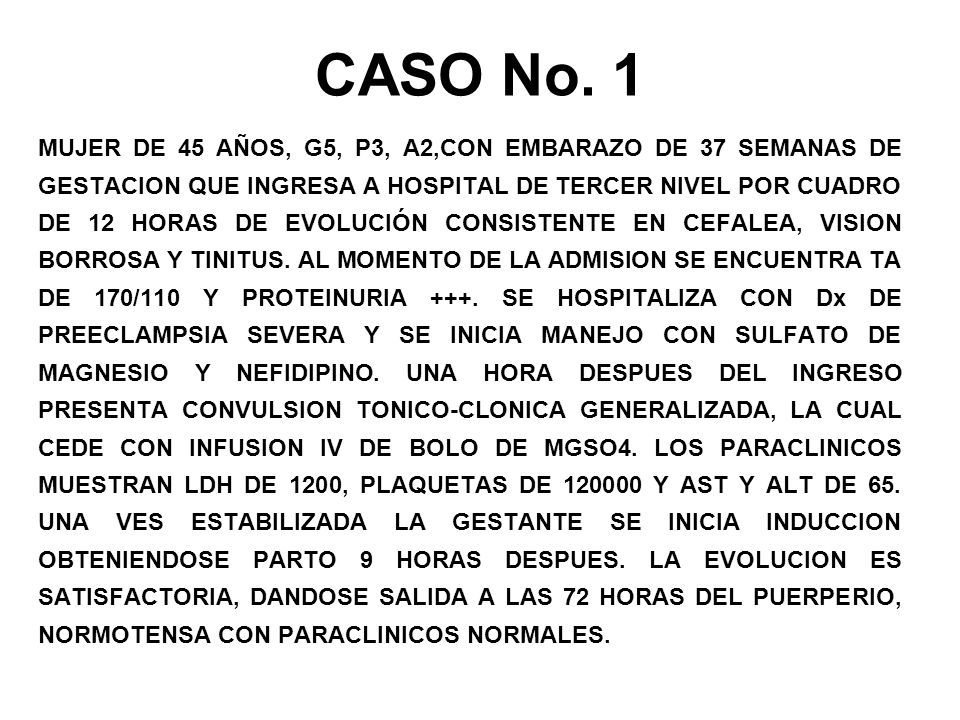The image consists of a block of text in Spanish, presented against a solid white background. At the top of the image in large, bold, black capital letters, the title reads "CASO NO. 1", indicating "Case Number 1". Below this title, the text is neatly left- and right-aligned, giving it an evenly spaced, justified appearance. The body of the text is composed of approximately 14 lines, all in smaller but still capital black letters. 

The content of the text appears to be a medical report focused on a 45-year-old woman, detailed as "mujer de 45 años, G5, P3, A2, con embarazo de 37 semanas de gestación," which translates to "a 45-year-old woman, G5, P3, A2, with a 37-week pregnancy." The report continues to describe her admittance to a tertiary-level hospital due to a condition evolving over 12 hours, marked by symptoms like headache, blurry vision, and tinnitus. The patient's blood pressure on admission is noted as 170/110, with a diagnosis supported by significant proteinuria. The detailed medical information suggests this text could be part of a clinical case report or examination documentation, shedding light on the medical condition and treatment considerations for this patient.